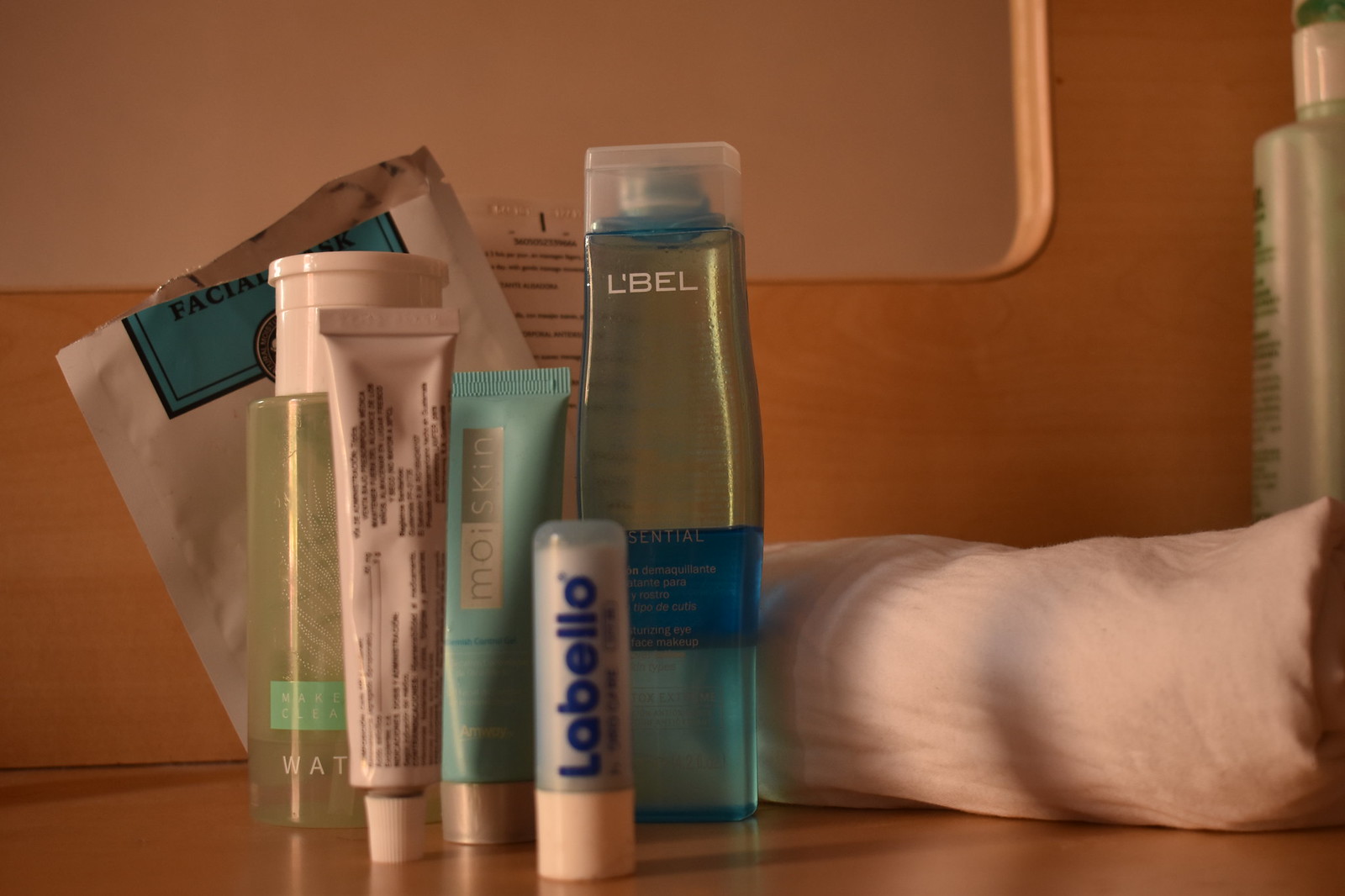The photograph captures a neatly arranged bathroom countertop, dominated by a wooden frame at the back which could either be the edge of a mirror or an open shelving unit. The surface is wooden, enhancing the warm, rustic aesthetic of the space. Scattered across the counter are various personal care items including an assortment of bottles and tubes. 

In the background, a ripped open paper packet, possibly containing foot soak or similar item, hints at recent use. In the foreground stands a clear bottle with something green inside, distinguishable by its white lid and green strip. Next to it, a tube turned backwards displays numerous small, unreadable writings and is capped with white.

Adjacent to this tube is a blue one labeled "Moiskin" in silver letters with a matching silver cap. In front of these items lies a tube of lip balm, clearly labeled "Labello" in blue letters against a clear bottle with a white cap. The largest bottle present is light blue with a clear cap, showcasing a dark blue band around two-thirds down its length, and the word "L-B-E-L" is prominently displayed in white near the top.

Additionally, a white cloth, seemingly rolled up, occupies the space next to the large bottle. Completing the scene, another large bottle—possibly shampoo—asserts its presence as the biggest item on the countertop. 

This meticulous arrangement paints a portrait of a thoughtfully organized bathroom scene brimming with everyday essentials.